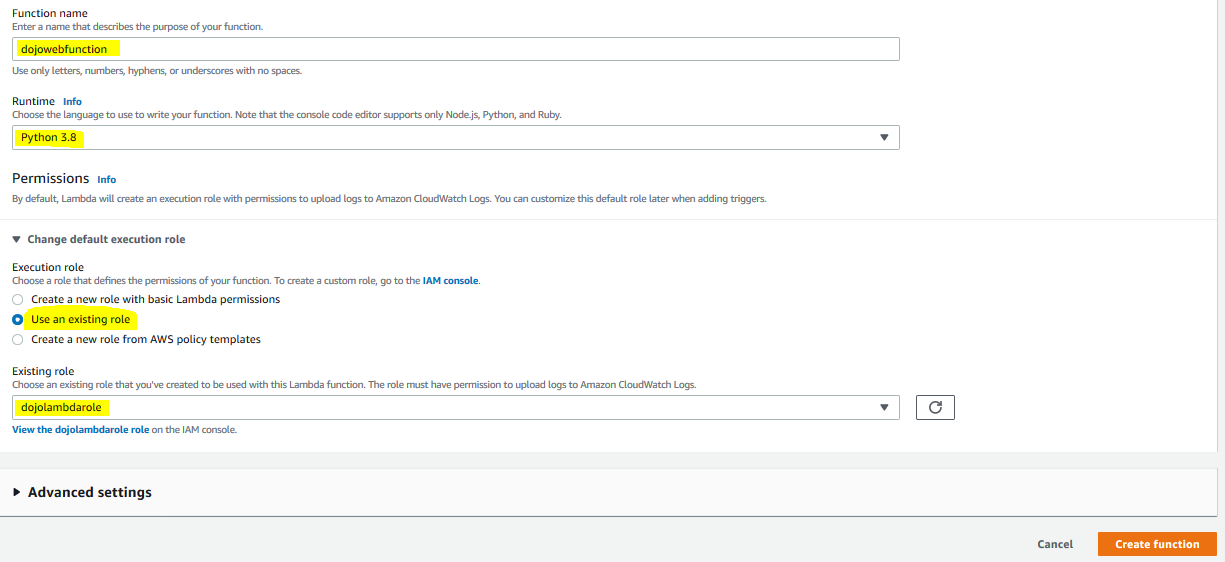The image displays a minimalist, web-based interface set against a stark white background. A thin gray border runs vertically along the left side of the screen, extending horizontally about two inches from the bottom edge. This border frames a small area which houses a right-pointing triangle icon adjacent to the text "Advanced Settings" in black font. Below this, the gray border resumes.

In the lower right corner, an orange tab labeled "Create Function" in white lettering is prominently featured, with a "Cancel" option in black text situated to its left.

At the top left of the interface, the section labeled "Function Name" in black instructs users to "Enter a name that describes the purpose of your function." This is accompanied by a rectangular input field. Further instructions below specify that only letters, common numbers, commas, hyphens, and underscores are accepted, without any spaces.

Continuing downward, the interface lists "Runtime" in black and "Info" in blue, paired with another input tab. Similarly, a "Permissions" section follows, with an accompanying blue "Info" label. Directly below, a drop-down tab labeled "Change Default Execution Row" appears under a line followed by the "Execution Row" label. 

On the left side, three circular icons are visible, with the middle icon shaded blue, while the others are white, each aligned with informational text. The section concludes with "Existing Row" and another line underneath, followed by a designated search area for user interactions.